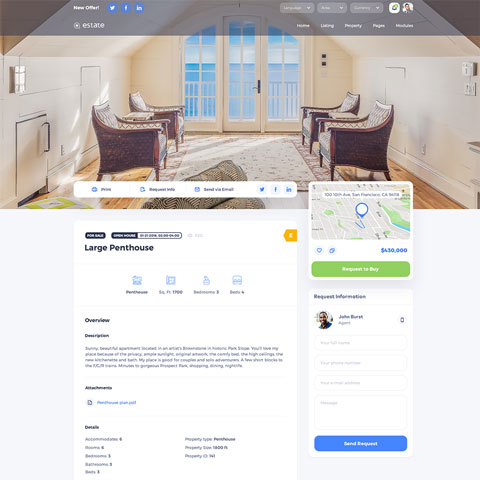**Image Description for Penthouse Listing**

The image features a cozy seating arrangement with four chairs placed on an area rug, positioned in front of elegant French doors. Despite the blurriness of the photograph, it offers a glimpse into the luxurious penthouse's living space. The listing provides an overview of the property details, including a spacious layout covering 1,450 square feet. This penthouse, listed at $430,000, boasts four bedrooms and three bathrooms.

For more information or to request details, potential buyers are directed to contact the agent, John Berg. The listing page also includes options to request additional information, send an email, or share the listing on Twitter. A map is provided to show the exact location of the property. 

Overall, the description emphasizes the expansive and upscale nature of the penthouse, encouraging interested parties to reach out for further details.